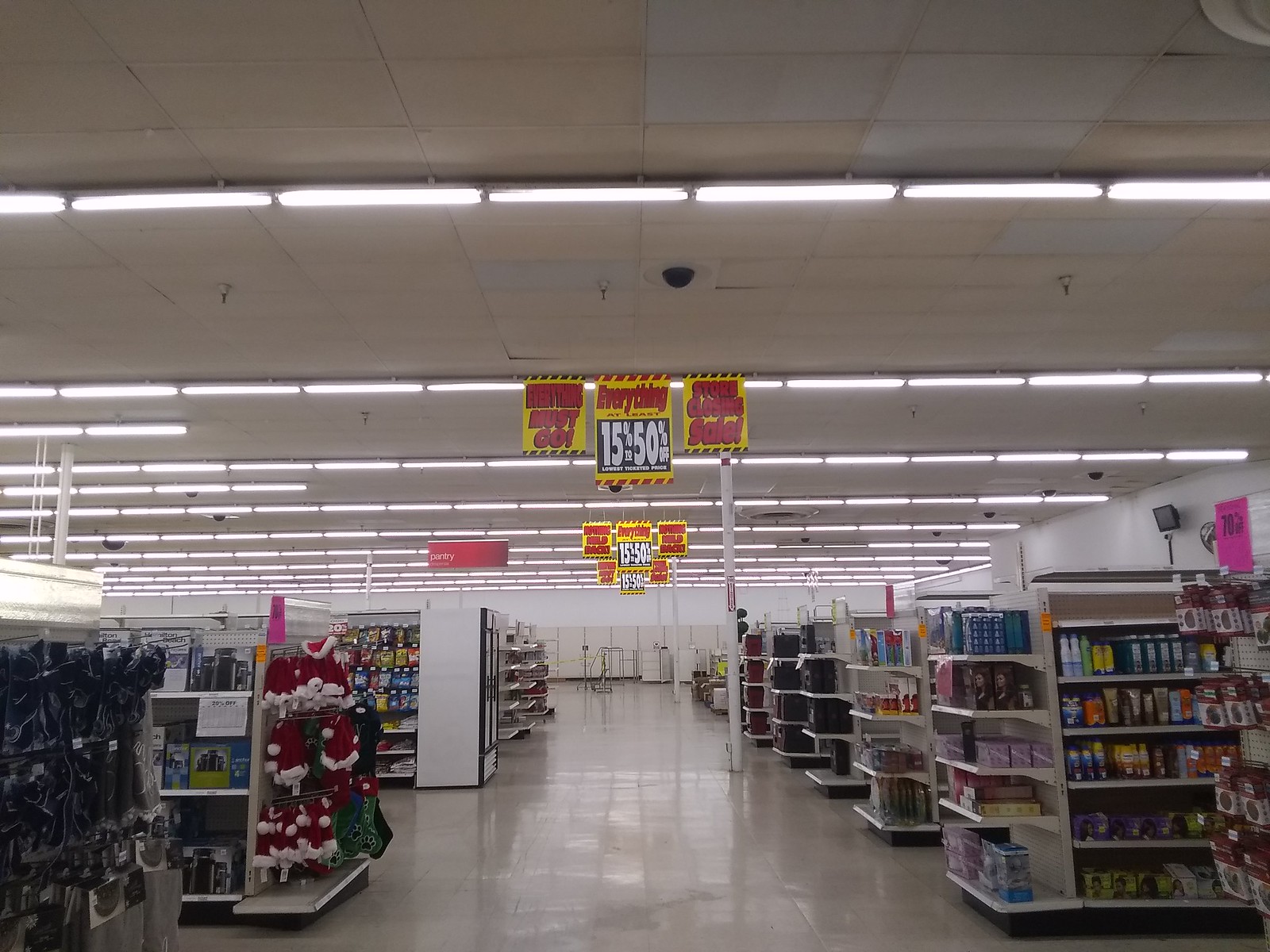This image captures the interior of a spacious, well-lit store, reminiscent of a Walmart or Kmart. The store features a white-tiled floor and white walls, amplifying the bright illumination from the many rows of closely spaced fluorescent lights on the ceiling. Prominent yellow sale signs with red lettering and black rectangles announcing discounts of 15% to 50% hang from the ceiling, indicating a major store closing sale. The shelves are densely stocked with a variety of items, including office supplies like papers, pens, and sunscreen. A noticeable section in the foreground is dedicated to hand creams, soaps, and lotions. Additionally, a vibrant display of Christmas hats adds a festive touch, with colors including red, yellow, blue, purple, orange, and green. Despite the visible abundance of products, some background areas appear emptier, highlighting the store's transitioning state.